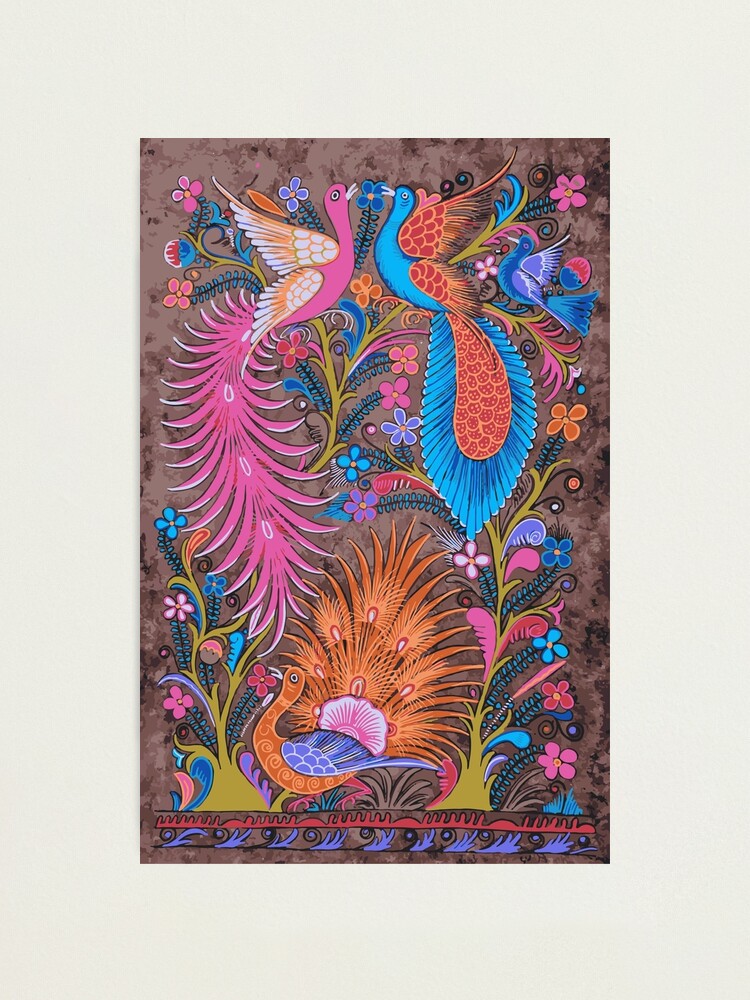This detailed piece of artwork, which appears to be painted or digitally created, is set against a beige to off-white background. The artwork itself has a patterned light brown backdrop adorned with darker brown swirls. The primary subjects are three brightly colored birds, each distinctly detailed. 

At the top left, there's a majestic pink bird with a long, flowing pink tail that stretches halfway down the image. It has orange and white wings, and its beak reaches toward a blue flower. To the top right is a striking blue bird with a shorter but fatter tail decorated with scalloped blue feathers around a large orange center. This bird features a vivid orange and red-dotted spot within its blue tail. Both of these top birds have their wings spread in a grand display, appearing to lean in for a kiss, creating a heartwarming centerpiece. Nestled between their wings is a very small, subtly detailed blue bird.

At the bottom of the artwork is a bird resembling a peacock, primarily orange with a grand orange tail and blue wings. This bird's tail feathers fan out and include white centers, reminiscent of a peacock's plume. It also has a small white beak, and it appears to be holding a pink flower.

Flanking these birds are two green plants or trees with vines stretching upward. These vines are adorned with an array of colorful, whimsical flowers, featuring hues of pink, blue, red, purple, and orange. The entire scene is vibrant and full of life, encapsulated within an off-white border that frames the intricate beauty of the birds and flowers.

This captivating artwork, with its blend of surreal birds and vivid plant life, might be showcased in an art gallery, commanding attention with its rich colors and detailed composition.